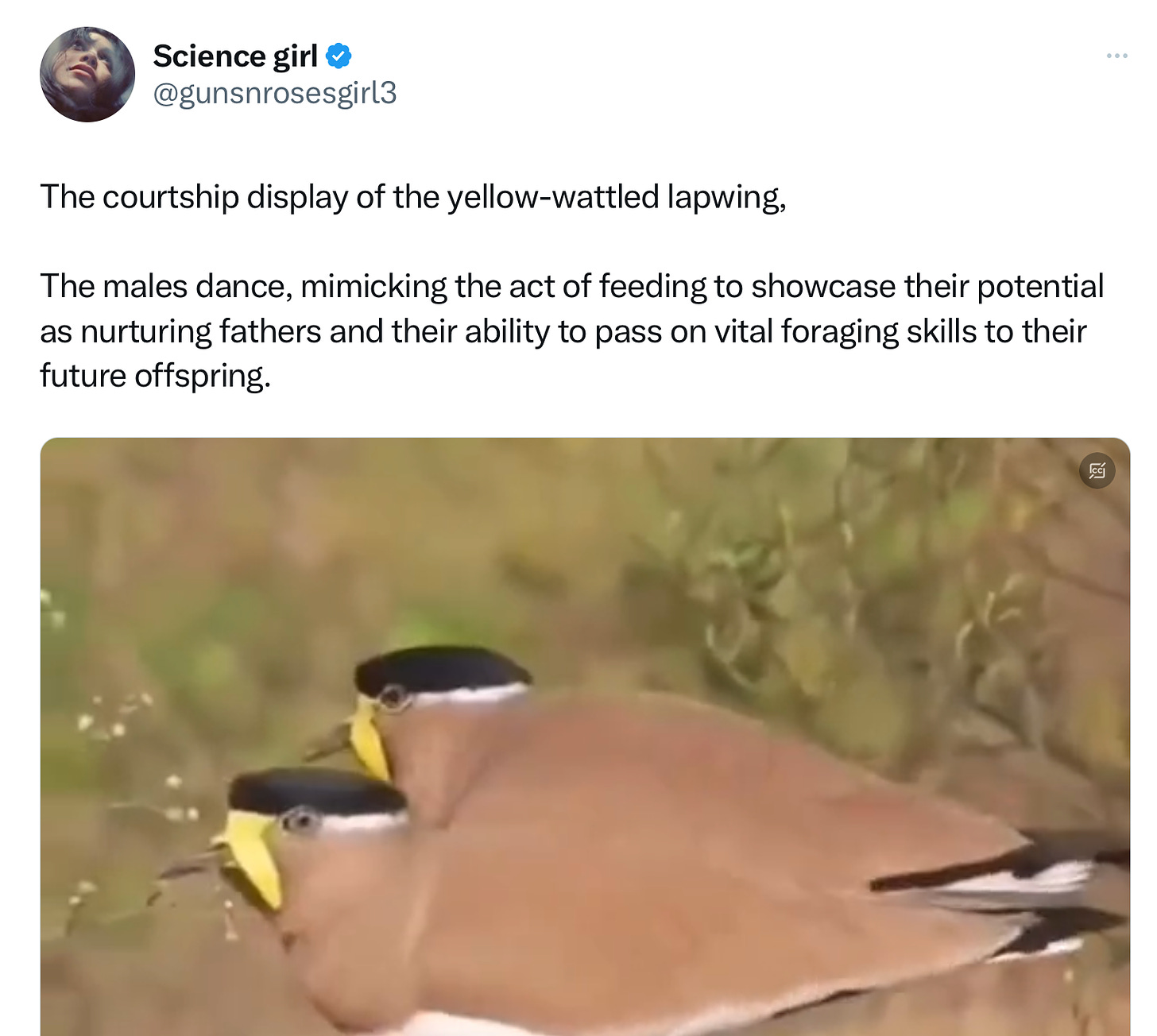This is a photograph of a tweet likely shared on social media. In the upper left-hand corner of the image, there is a circular profile picture of a young woman looking up, accompanied by her name "Science Girl" along with a blue checkmark and the handle "@GunsNRosesGirl3." Below her name, the tweet reads: "The courtship display of the yellow-wattled lapwing. The male's dance mimicking the act of feeding to showcase their potential as nurturing fathers and their ability to pass on vital foraging skills to their future offspring."

Directly underneath the text, there is a wide horizontal rectangular image depicting two yellow-wattled lapwing birds. They appear to be perched on a twig against a blurred background with hints of brown and green. The birds are sitting side by side, facing left. They feature distinctive characteristics: brown bodies with white undersides, black flat tops on their heads adorned with a white ring around them, and prominent yellow beaks extending from yellow facial markings. Their tails are black with white accents beneath, and the detailed portrayal almost gives the impression that they are two heads emerging from the back of a filleted chicken breast laid on a surface. This visual peculiarity adds a unique touch to the photograph, making it seem as if the birds are blowing bubbles and bringing to mind a fascinating resemblance to Siamese birds crafted from a chicken breast.